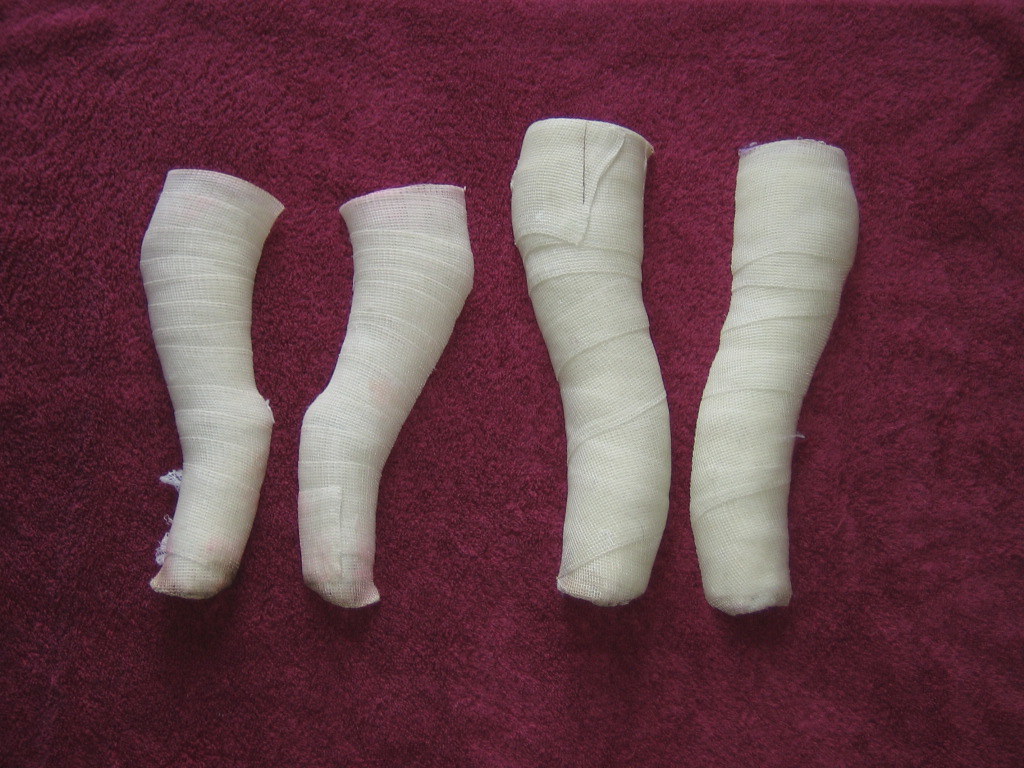The photograph captures four white plaster casts arranged on a dark maroon, low-pile carpet. These casts appear to be orthopedic molds likely used for immobilizing limbs. The two on the left are slightly smaller, distinctly shaped to resemble feet standing en pointe, potentially for the legs of a small person. The pair on the right are larger with a less defined foot shape, possibly crafted for arms. All four casts exhibit textured bandages, indicative of traditional plaster wrapping techniques. The consistent alignment and bandaging details underscore their purpose while highlighting the stark contrast against the rich, dark maroon carpet.